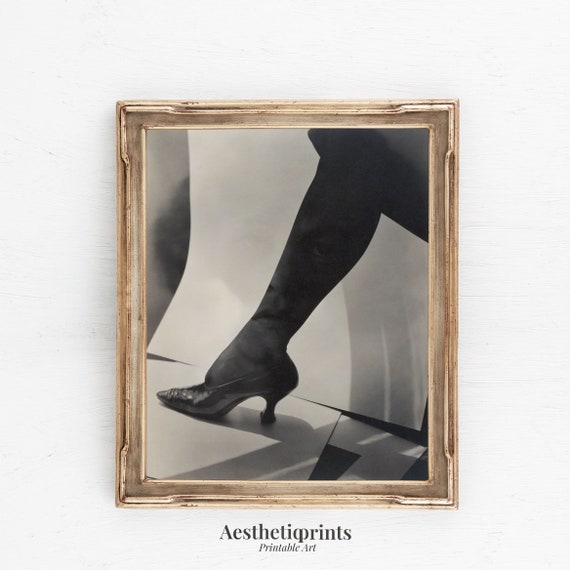This image showcases an art piece in a rustic, light, and dark brown wooden frame mounted on a white wall. The artwork itself appears to be a black-and-white photograph featuring the close-up of a woman's leg adorned in black pantyhose and a black high-heeled shoe. Captured in a stark, monochromatic palette, the leg is positioned against a white floor with a black corner in the bottom right, and a white wall with a small black section on the left. The woman’s other leg is either suggestively crossed above the visible one or represented by a shadow or outline that gives an impression of a large skirt. Additionally, there is an intriguing reflection or design element superimposed on the image that resembles a face. Below the photograph, the text "aesthetic prints" is prominently displayed in bold letters, with "printable art" in smaller, black letters underneath. The rustic frame and minimalist composition contribute to the piece's overall aesthetic appeal.